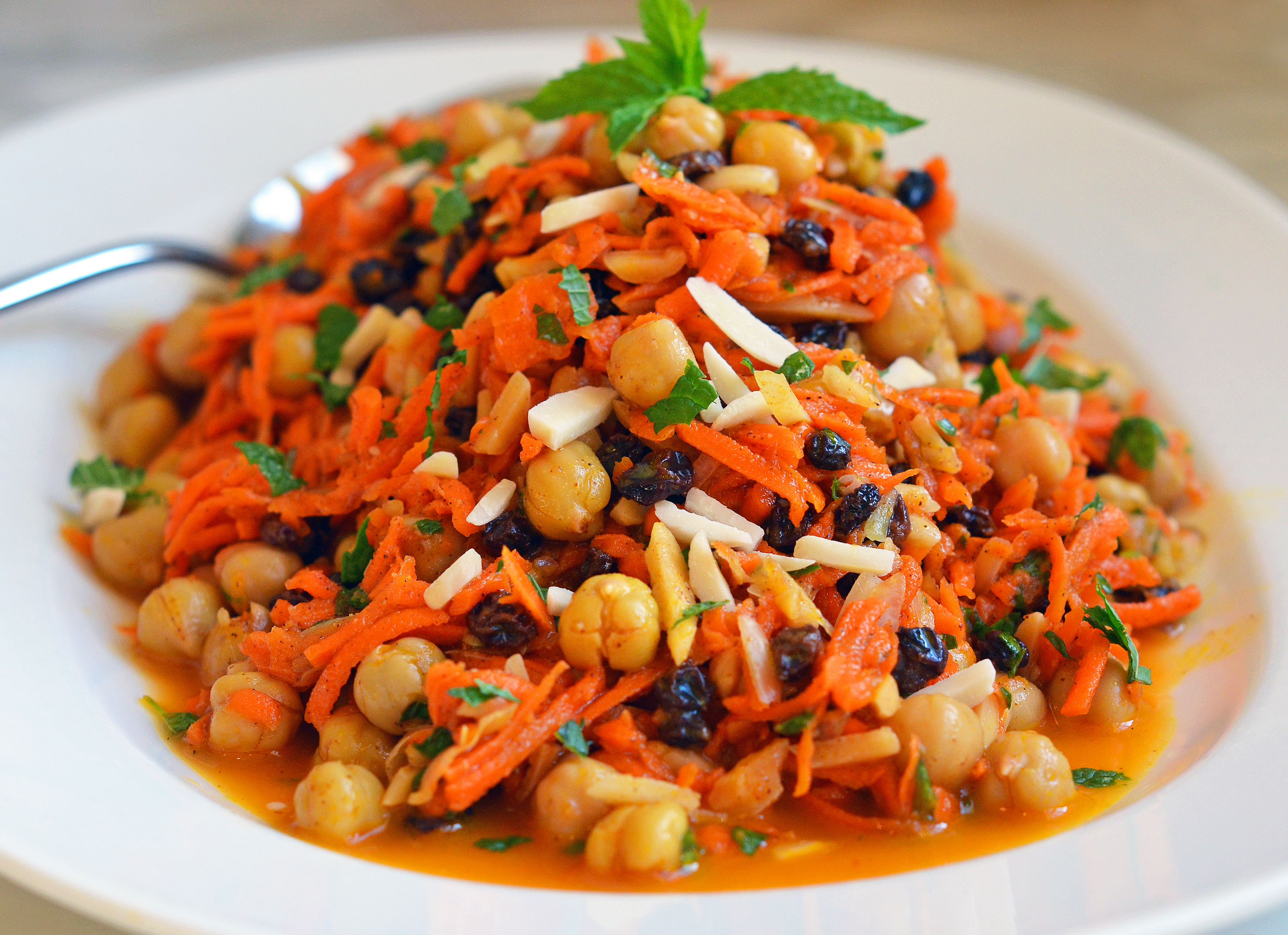The image depicts a vibrant vegetable and bean salad presented on a large white plate placed against a brown background. A silver spoon rests on the left side of the plate. The salad itself is a colorful medley featuring chickpeas, julienned shredded carrots, raisins, and possibly a mix of garbanzo and black beans. Additionally, there are water chestnuts and small amounts of cheese interspersed throughout the dish. The salad is nestled in an orange, juicy sauce or broth. Green herbs, such as basil, are finely cut and add additional texture and color. The entire mound of the salad is crowned with a fresh mint sprig, adding a touch of elegance to the hearty dish. The photograph captures the salad in sharp detail while the edges remain slightly hazy, focusing attention on the dish's contents.